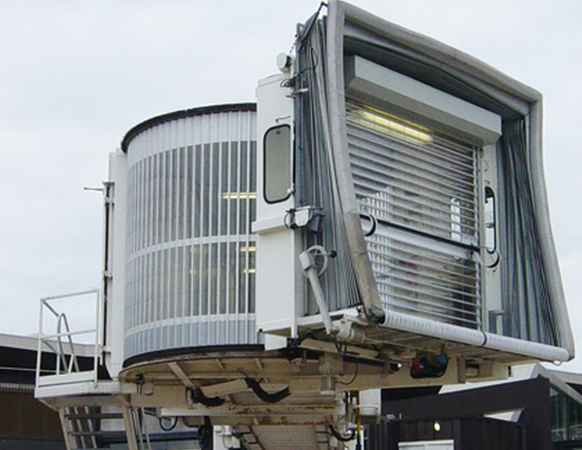The image depicts a large, metal jet bridge primarily centered in the frame, although it leans slightly to the right when considering the attached staircase. The structure is essential for connecting an airplane to the terminal, allowing passengers to board and deboard safely without exposure to the elements. It features a cylindrical body with light blue, white, black, and gray colors, accented by a light brown hue. Vertical slats are visible on the cylindrical segment, while horizontal grates are present on the side section that attaches to the plane’s door. There is a set of metal stairs on the far left leading up to the entrance. The setting is industrial and workplace-oriented, likely situated on an airport tarmac. The object is well-lit from the inside, illuminating the structure and highlighting its use as a functional and mobile workspace in aviation settings.